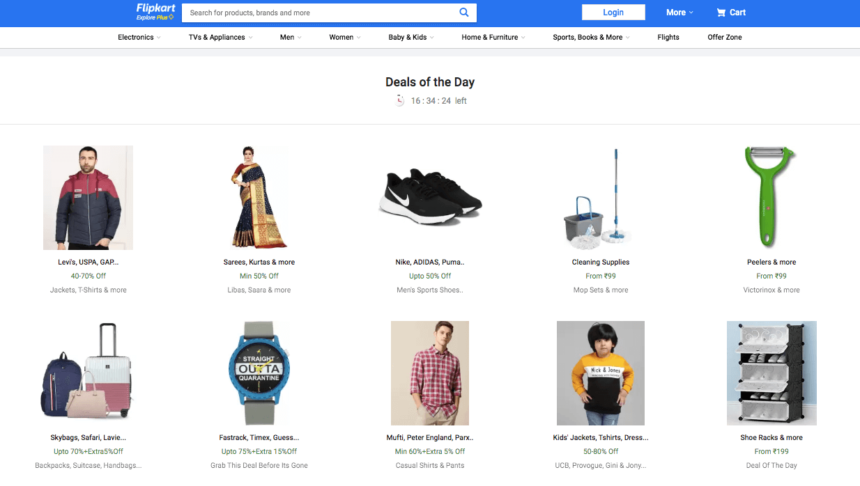This screenshot captures a web page from the popular shopping site Flipkart, viewed on a desktop computer. The recognizable Flipkart logo, featuring the word "Flipkart" in white, is situated on a blue navigation bar at the top left of the screen, adjacent to a search menu. To the right of the search menu, the interface displays buttons for Login and More options, along with a shopping cart icon.

The main content begins with a prominent header on a white background reading "Deals of the Day," showcasing the day's highlighted deals. Below this header, the page is organized into a grid layout, featuring 10 products. These products are displayed in two distinct rows, each containing five items, making navigation and comparison straightforward for the user.

Each product entry includes an image accompanied by a brief description. Specifically, in the top row, at the very center, there is a clear image of a pair of black and white Adidas sneakers, catching the eye with its stylish design. This meticulous arrangement and detailed presentation facilitate a user-friendly shopping experience.